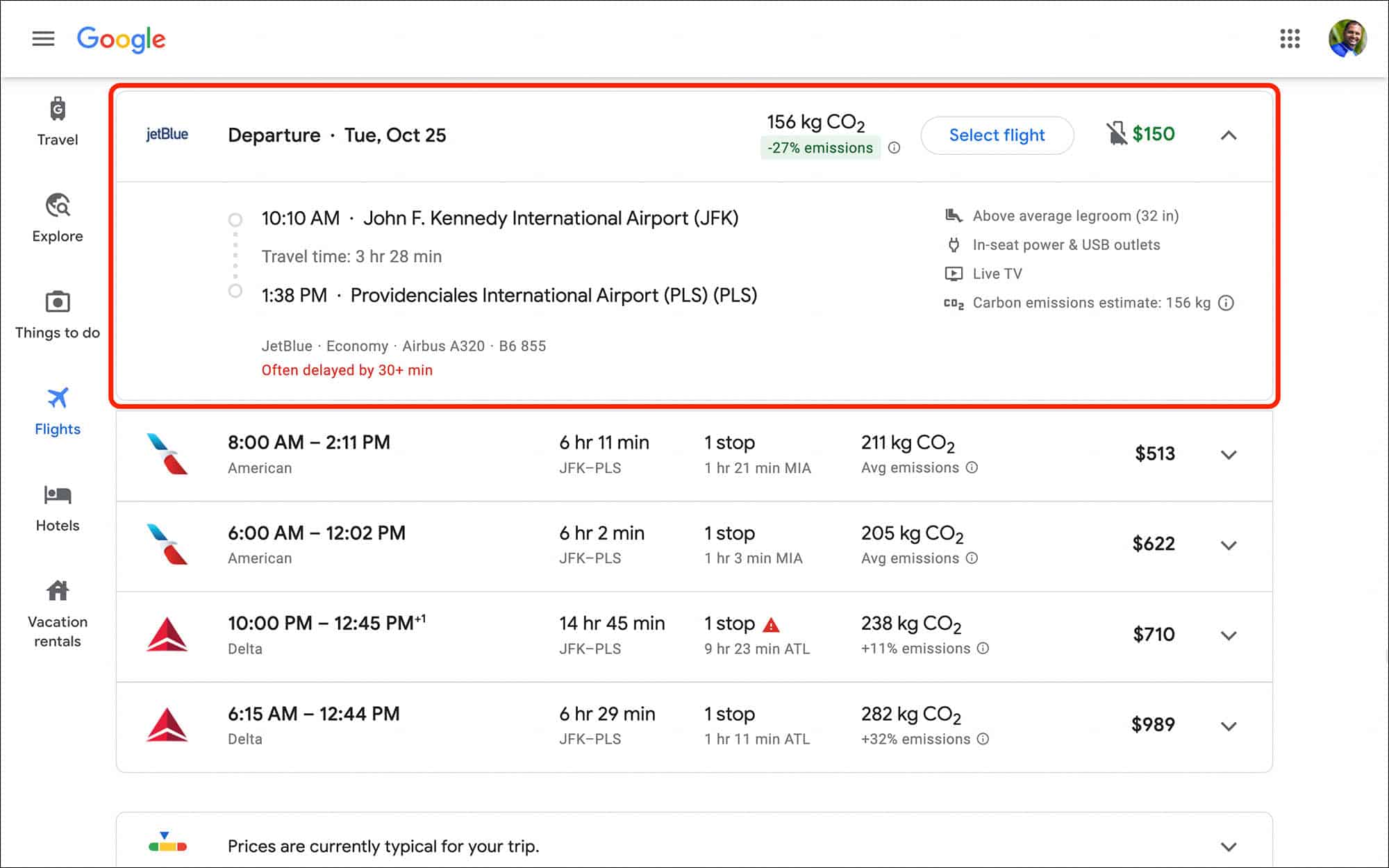Here is an enhanced and detailed caption for the described image:

---

This image is a screenshot featuring a clean white background bordered by a thin gray line. At the upper left corner, the text "Google" is displayed, and at the upper right corner, there's a small, circular profile image of an individual with dark hair, wearing a blue and white shirt—though the gender is not clearly identifiable.

Prominently outlined in red is a rectangular area with the heading "JetBlue." The details within this section indicate a departure scheduled for Tuesday, October 25th, including an environmental impact note of "156 kg CO2" displayed in a green box, signifying a "negative 27% emissions." To the right of this information is a clickable option labeled "Select flight" in blue text. Adjacent to this, an icon depicting a suitcase with a diagonal slash through it indicates a baggage fee of "$150."

Detailed flight information is provided below: The departure time from John F. Kennedy International Airport (JFK) is listed as "10:10 a.m.," with an estimated travel duration of "3 hours 28 minutes." The arrival time is noted as "1:38 p.m." at Providenciales International Airport (PLS). The flight service is offered by JetBlue, operating an Economy class seating on an Airbus A320 aircraft.

---